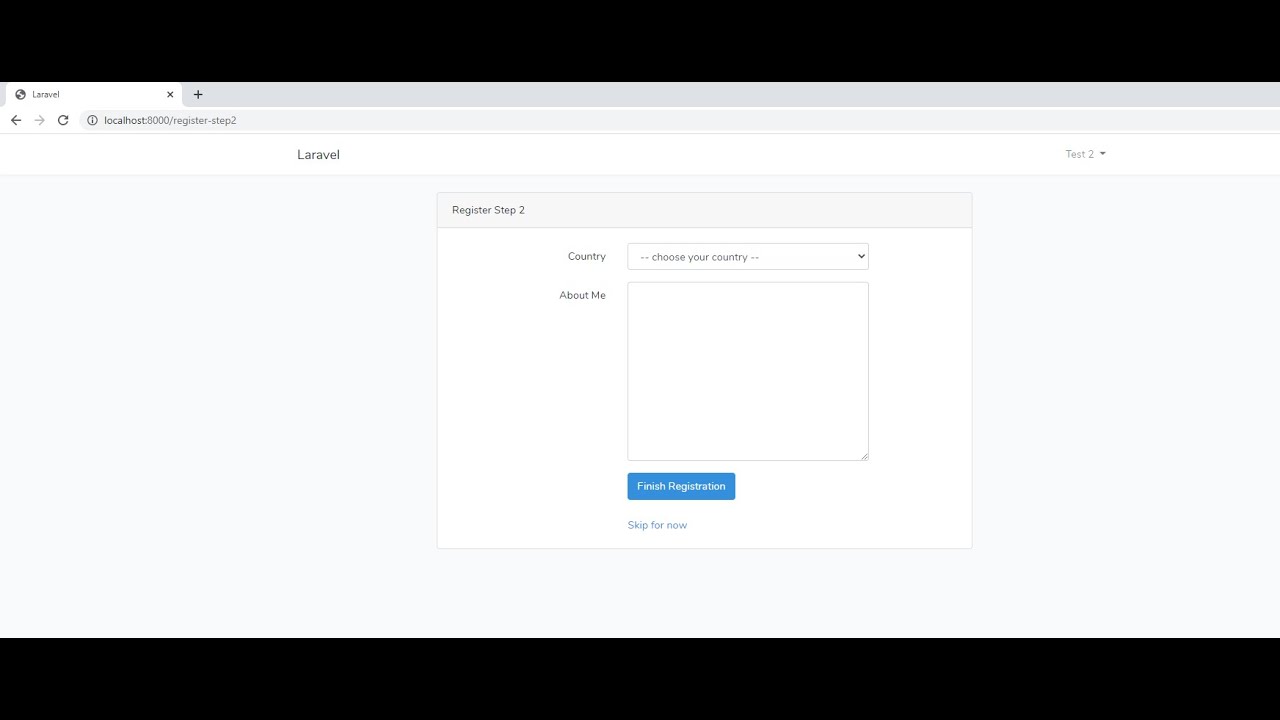The image depicts a web page, accessible via the URL "localhost:8000/register-step-two." At the top of the page, the title "Laravel" is displayed, and in the upper right-hand corner, there is a label "test2" accompanied by a downward-pointing arrow. The main content area features a heading titled "Register Step Two."

Beneath this heading, there is a form section starting with a label "Country" followed by a dropdown menu prompting the user to "Choose your country." Below this dropdown, there is another section labeled "About Me" with an input box where users can write additional information about themselves. 

At the bottom of the form, there is a prominent blue button labeled "Finish Registration." Directly below this button, there is an option "Skip for now" in plain text. The entire web page has a clean white background.